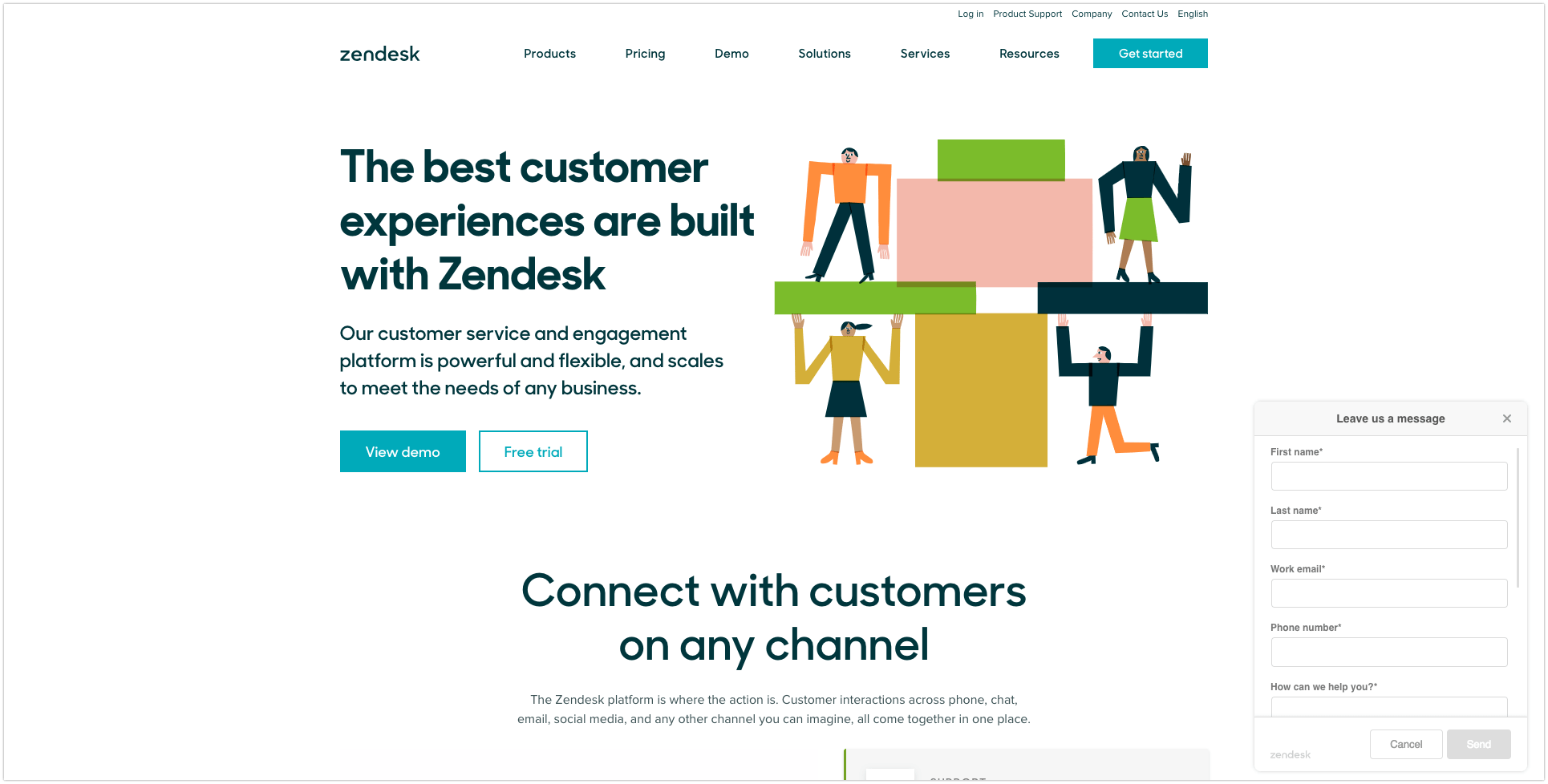The image displays the home page of Zendesk's website. At the very top, the company's name "Zendesk" is prominently featured, accompanied by several navigation options: Products, Pricing, Demo, Solutions, Services, Resources, alongside a blue "Get Started" button. Additional buttons like "Login," "Product Support," "Company," "Contact Us," and a language selection indicating "English" are also visible.

Dominating the center of the page, a bold statement reads, "The best customer experiences are built with Zendesk," emphasizing the capabilities of Zendesk's customer service and engagement platform. This statement is supported by subtext that describes the platform as powerful, flexible, and scalable to meet the needs of any business. Below this text are two call-to-action buttons: a blue "View Demo" button and a white "Free Trial" button.

The foreground features an artistic depiction of diverse characters with exaggerated long arms standing on box-like structures, adding a whimsical touch to the page. Lower down, the page highlights a key feature of the Zendesk platform: "Connect with customers on any channel," elaborating that Zendesk consolidates customer interactions across phone, chat, email, social media, and other channels into a unified interface.

A contact form is also present, inviting visitors to leave a message with fields for First Name, Last Name, Work Email, Phone Number, and a question about how Zendesk can assist them. The form includes "Cancel" and "Send" buttons for user convenience. The overall design of the page is clean, featuring a white background with black text.